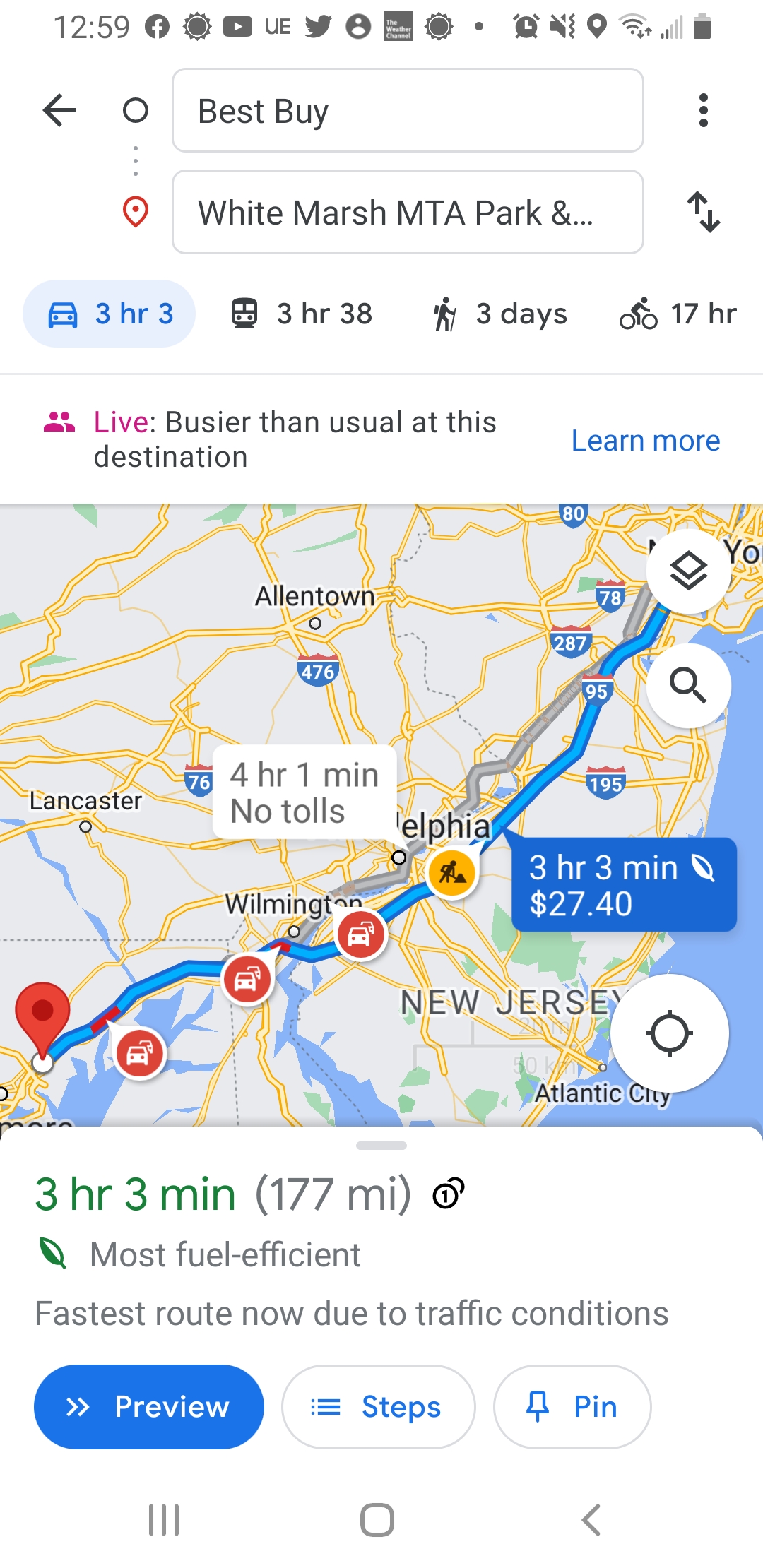This is a detailed screenshot of Google Maps directions displayed on an Android smartphone. At the top, the interface shows white boxes for the starting location, Best Buy, and the destination, White Marsh MTA Park. The current time is 12:59 p.m., indicated in gray text in the upper left corner. Also visible are various icons representing other running apps, battery life, and cellular signal strength. Below the destination information, the map provides estimated travel times: 3 hours and 3 minutes by car, 3 hours and 38 minutes by bus, 3 days by walking, and 17 hours by bicycle.

The map itself highlights a recommended route shown with a blue line, spanning from York, Pennsylvania, through Wilmington, Delaware, and onward. Major highways and state borders, including New Jersey and Atlantic City, are visible. The route is marked as the most fuel-efficient and fastest option due to current traffic conditions.

Additionally, a note reading "Live busier than usual" at the destination is visible, with an option to learn more in blue text. The route time of 3 hours and 3 minutes covers 177 miles, and there are other route options shown, including a toll-free route taking 4 hours and 1 minute. Information regarding a toll amount of $27.40 and three red signs that may indicate traffic accidents are also noted.

At the bottom, three oval-shaped buttons labeled "Preview," "Steps," and "Pin" are displayed, alongside the Android interface buttons.